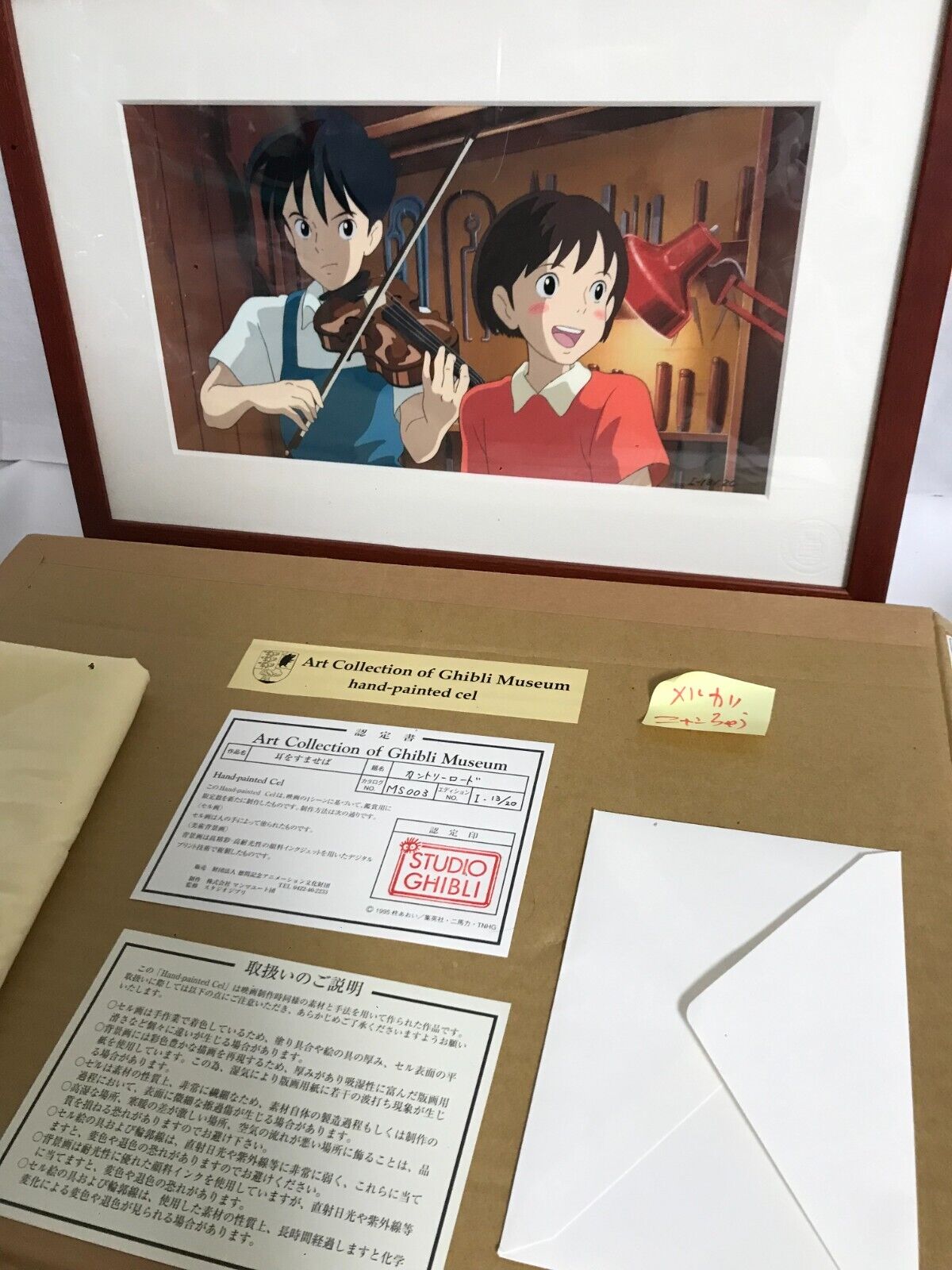This photo showcases a detailed display centered around a framed animation still from a Studio Ghibli film, likely set in a workshop or garage. The framed image features a boy with black short hair, wearing a white shirt with overalls, playing the violin. On his right, a girl with short brown hair, blush on her cheeks, a smile on her face, and a white blouse with a Peter Pan collar under a red top looks away from him. A red desk lamp and various tools are visible in the background, enhancing the workshop ambiance.

In front of the framed picture, resting on what appears to be a cardboard surface, is a collection of certificates and documents related to the artwork. A yellow piece of paper prominently states "Art Collection of Ghibli Museum Hand-Painted Cell," accompanied by a Studio Ghibli-stamped certificate and another document filled with Japanese text. To the right of these papers, there is an envelope and a sticky note with Japanese characters. On the left side of the display, partially out of view, lies a folded piece of cloth. The entire setup hints at the meticulous certification and presentation of the animation cell, emphasizing its authenticity and connection to the Ghibli Museum.